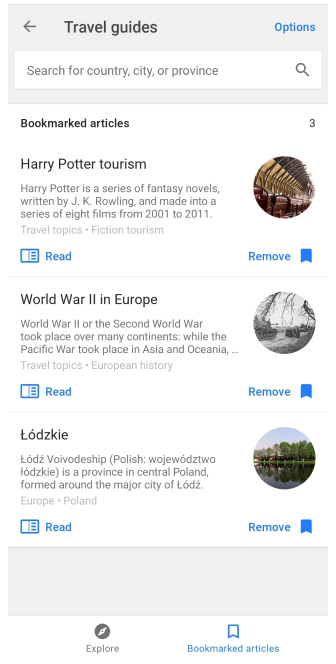In the image, the top-left corner features the text "Travel Guides" in black. To the left of this text, there's a left-pointing arrow resembling a backspace arrow. On the top-right, the word "Options" appears in light blue. Below the "Travel Guides" text, a search bar is positioned, containing the placeholder text "Search for country, city, or province," with a magnifying glass icon on the far right of the bar.

Beneath the search bar, three sections labeled "Bookmarked Articles" are visible:

1. The first article is titled "Harry Potter Tourism." Below the title, it indicates, "Harry Potter is a series of fantasy novels written by J.K. Rowling and made into a series of eight films from 2001 to 2011." A circular profile picture, resembling a train, is located to the right of the article snippet.

2. The second article is titled "World War II in Europe." It briefly explains, "World War II or the Second World War took place over many continents, while the Pacific War took place in Asia and Oceania." This article also has a profile picture positioned to the right of the text.

3. The third article is titled "Łódź, Łódzkie" and explains, "Łódź, a province in central Poland, is formed around the major city of Łódź."